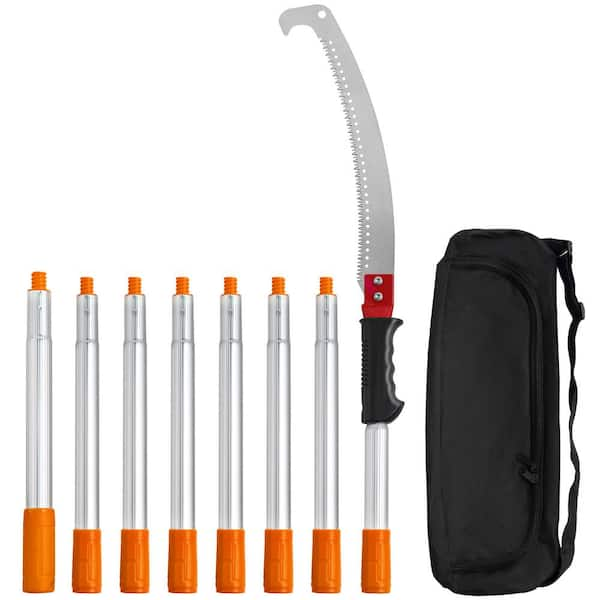The image depicts a professionally photographed set of eight tubular tools positioned vertically against a white background. Each tool has three distinct components: an orange base handle, a metallic silver or perhaps clear plastic tubular middle section, and an orange screw-like top. The tools vary slightly in height, with the tallest on the far left and possibly the shortest on the far right. The tool on the far right is unique as it features a small saw attachment. This saw has a black handle extending halfway down the silver tube, transitioning to a red segment with two silver rivets, and a saw blade with teeth on the left side that curves slightly. To the far right of the arrangement lies a black, portrait-oriented bag crafted from heavy cloth with a strap running its length and a zippered section on the side. This bag is presumably designed to store the tools. The saw attachment possibly functions as an extension for cutting tasks, such as trimming branches on tall trees.